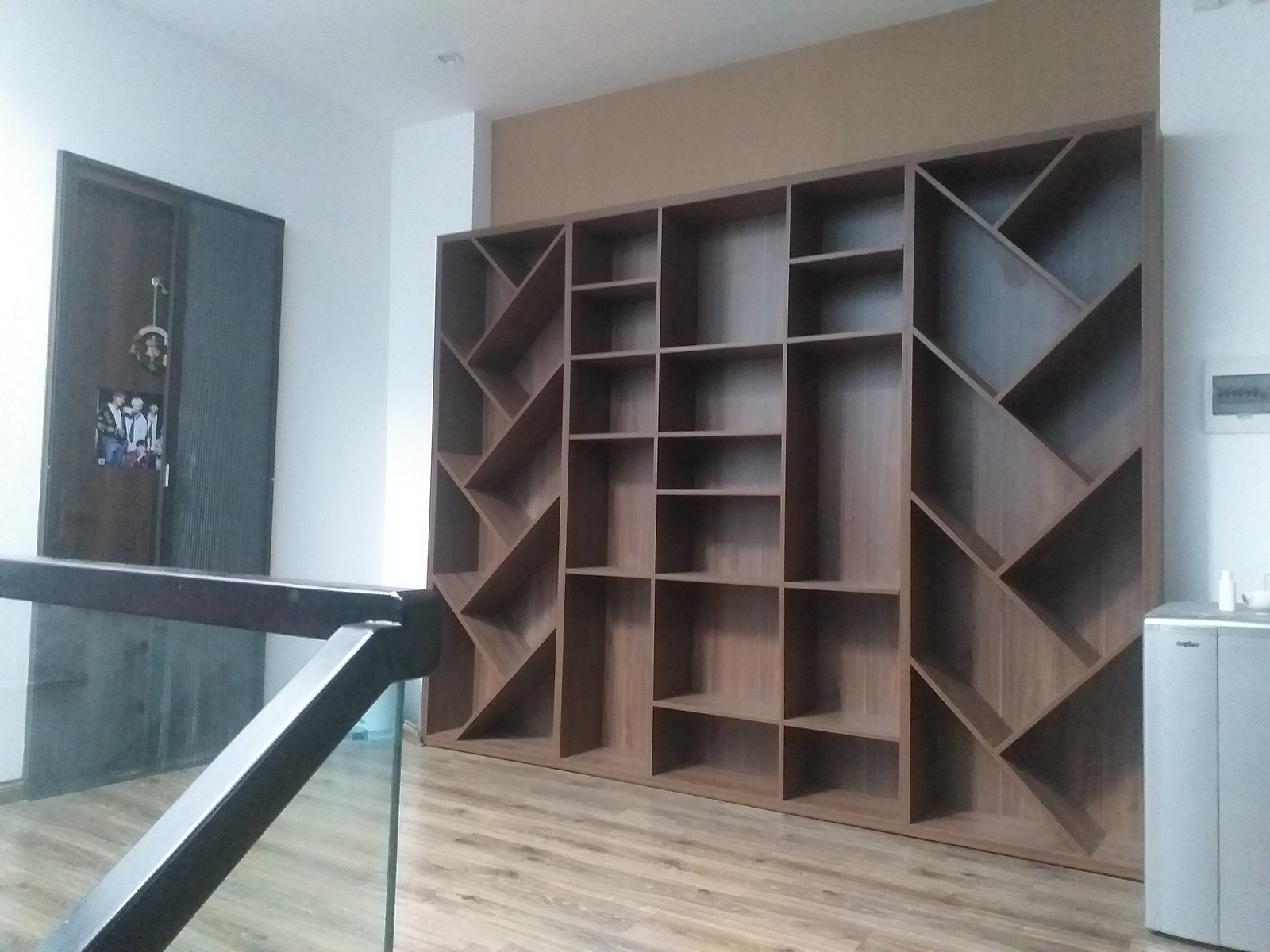The photograph is a vibrant, landscape-format image showcasing a unique indoor space with a prominent bookshelf. Taken from a slightly lower vantage point on a staircase, the image reveals a hallway or landing area adorned with modern design elements. To the right, a mounted stainless steel water faucet and a vent are visible on the wall. The stairs, featuring a plexiglass barrier with a silver trim and handrails, lead up to the first floor, enhancing the contemporary aesthetic.

Dominating the back wall is an eye-catching wooden bookshelf in a deep brown color. The central section of the bookshelf is traditional, with horizontal shelves at various heights forming conventional compartments. However, the sections on either side introduce a striking variation: the shelves are slanted at different angles, creating dynamic triangular and rectangular spaces, with some forming shapes resembling the letter "Y." This inventive design adds visual interest and practical versatility.

On the left side of the image, a doorway with a glass panel includes a picture of people, and a nearby white-painted wall hosts a hanging picture and a small decorative item. The wooden flooring ties the elements together, grounding the space in warmth and sophistication. The overall scene captures a harmonious blend of functionality and artistic design in a residential setting.